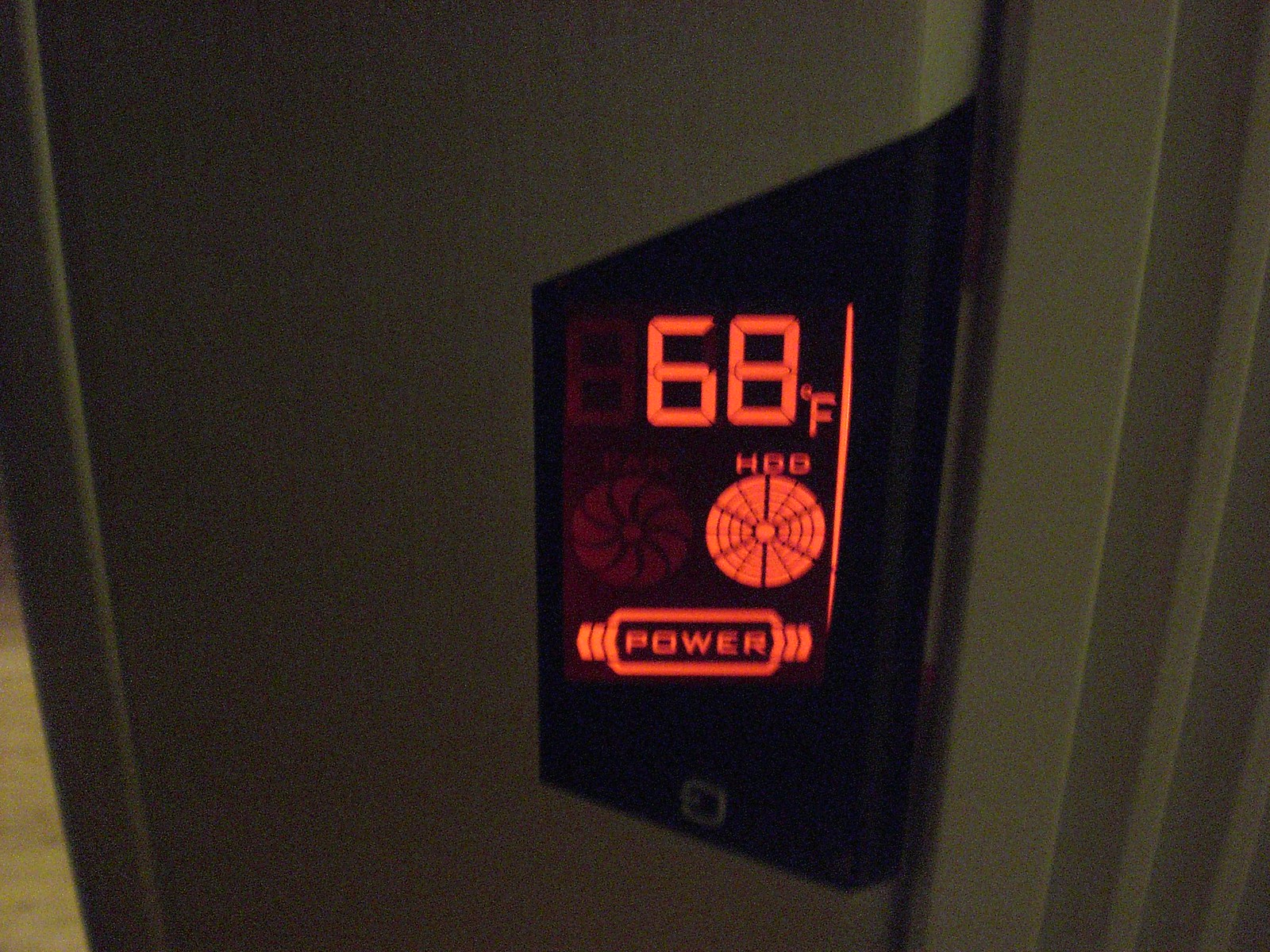This detailed close-up photograph showcases a dark gray structure with a subtle greenish tint, initially suggesting it might be a wall or door. However, upon closer inspection, the image features a trapezoidal screen, tilted on its side, at its center. This screen displays information in a light red font reminiscent of analog clock text. Dominating the top of the screen are the large red numbers "68°F", likely indicating temperature in Fahrenheit. Directly beneath this, a fan icon is marked with the letters "HDD". Further down, a larger rectangular icon with arrows pointing outward is labeled "Power". Below these icons and text, there is an additional button or dial. The intricate details suggest this structure is not merely a wall or door but a control panel or interface for a device, providing essential operational data and controls.